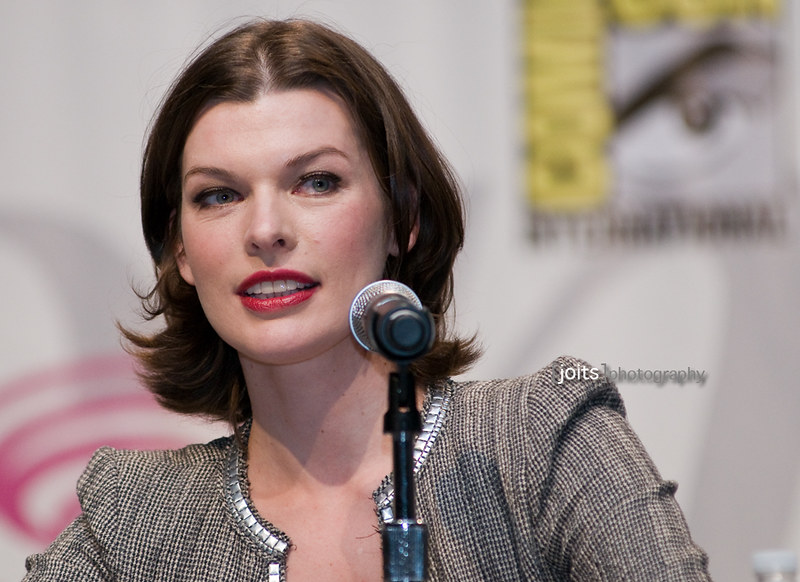This photograph features Milla Jovovich, a popular actress, engaging in a speaking event at Comic-Con in San Diego, as indicated by the visible Comic-Con International logo in the background. She has shoulder-length brown hair that curls slightly upwards at the ends, and she is wearing a dark brown jacket or shirt. With delicate facial features accentuated by striking bright red lipstick, her appearance is notably elegant yet slightly surprising due to the vivid lip color. She is positioned in front of a microphone, clearly engaged in a speaking role, likely part of a panel discussion about films or television shows. Above her shoulder is a watermark reading "joits Photography" with "joits" in white and "Photography" in gray. The overall setting appears to be brightly lit with a typical white background, suggesting this image is from the early 2000s when such themes were common at Comic-Con events.